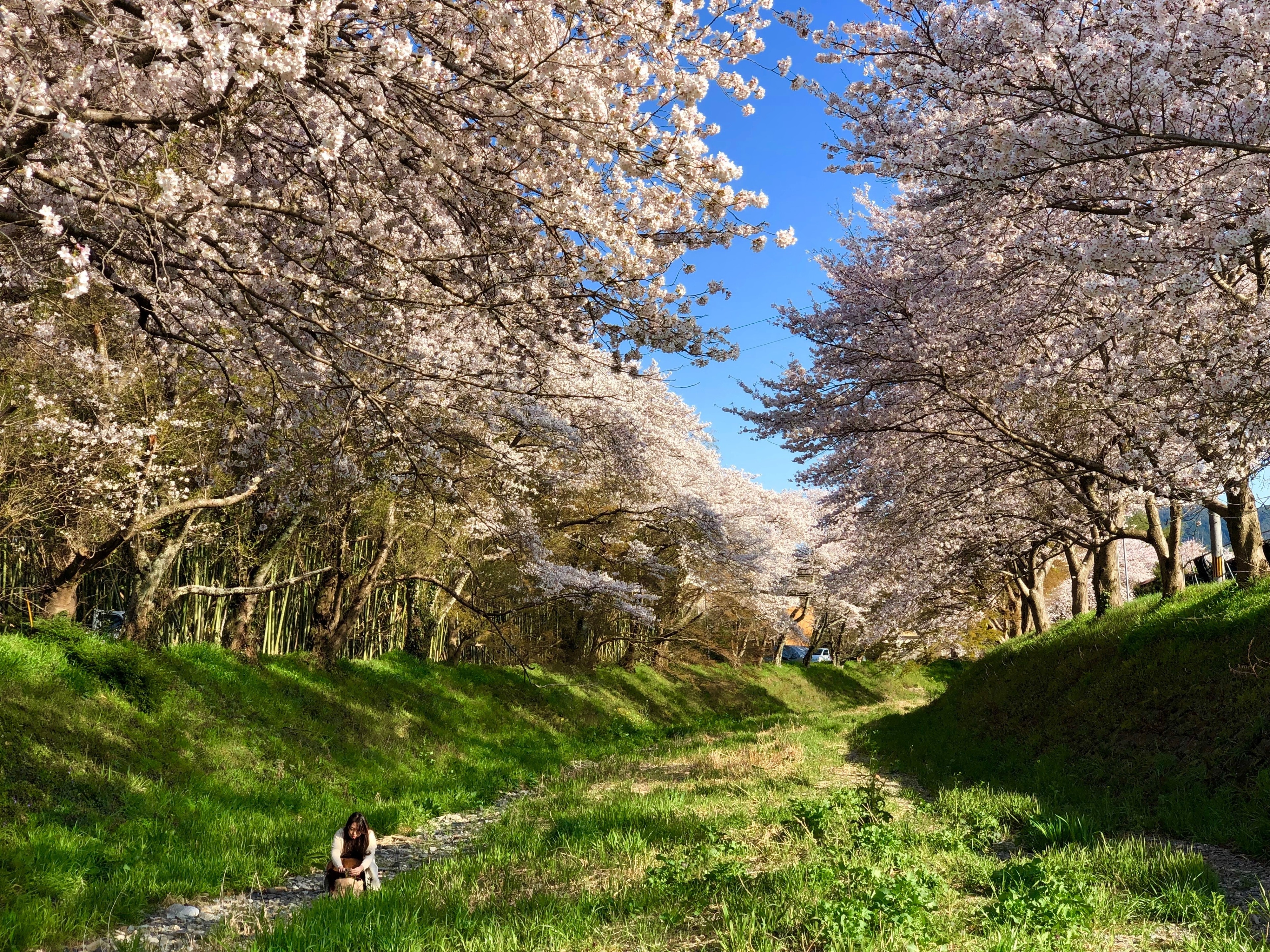A picturesque photograph captures a serene springtime scene in a lush, green valley nestled between two gentle hills, each adorned with tightly-packed cherry blossom trees in full bloom. The cherry trees, with their delicate pinkish-white blossoms contrasting against their brown trunks, line the slopes of the hills, creating a natural frame for the sparkling blue sky that peeks through at the top of the image. The valley floor is carpeted with bright, vivid green grass and intersected by a man-made rocky path or stream bed. In the foreground, a woman with dark straight hair, dressed in white clothing, is crouched down on some stones, intently focused on an object in her hands. She is positioned towards the camera but looking downward, adding a human element of quiet contemplation to the tranquil landscape. In the background, beyond the serene cherry trees, a few cars are visible, hinting at the world beyond this peaceful haven.